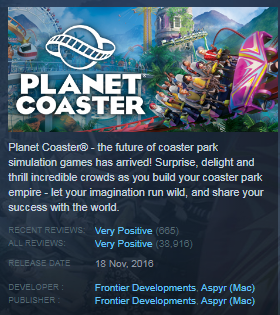The image showcases a vibrant and cartoonish portrayal of a planet-themed roller coaster park. At the center, a spherical planet is prominently featured with a roller coaster track wrapping around it, symbolizing the global thrill of this amusement experience. The sky is depicted in shades of gray and blue, adding a dynamic backdrop to the lively scene below.

Numerous roller coaster tracks crisscross the image, contributing to an atmosphere of excitement and adventure. In the background, a building can be seen with patches of moss, set against a picturesque landscape of hills and mountains.

A striking purple roller coaster car, adorned with lines and perhaps some seeds, adds a splash of color to the scene. The overall image exudes energy and anticipation, inviting viewers to imagine the thrills that await.

Text accompanying the image proudly introduces "Planet Coaster," declaring it the future of coaster park simulation games. The game invites players to delay and thrill incredible crowds while building their coaster park empire, encouraging imagination and sharing success with the world.

Highlighted are very positive reviews: 665 recent reviews and a total of 38,916 reviews, underscoring the game's popularity. The release date is noted as November 18, 2016, developed and published by Frontier Developments and Asper, with Matt specifically mentioned in parentheses.

The background of the image presents a grayish hue, providing a neutral canvas that accentuates the detailed and imaginative elements of the Planet Coaster scene.